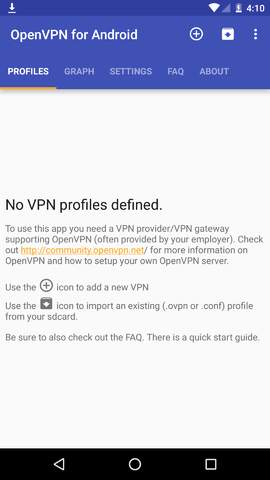This image captures a screenshot of a site, specifically an app interface. At the very top, there's a thin, darker blue banner featuring an arrow pointing downwards with a line underneath it. Moving to the right, the banner displays icons for the Wi-Fi signal, cell signal, and battery status, which reads "410."

Below the dark blue banner, there is a lighter blue-purple section with the text "OpenVPN for Android" in white, with "VPN" prominently capitalized. This section also contains a navigation bar with a circle containing a plus sign, a square with a downward arrow, and three vertical dots.

Underneath this section, several navigation options are listed in all capital letters: "PROFILES," "GRAPH," "SETTINGS," "FAQ," and "ABOUT." "PROFILES" is highlighted in bold white print and underlined in orange.

Moving further down to a white background, there's a bold-text notification that reads: "NO VPN PROFILES DEFINED." The text continues by explaining, "To use this app, you need a VPN provider/VPN gateway supporting OpenVPN (often provided by your employer)." It then instructs users to visit a website for more information on OpenVPN and how to set up their own OpenVPN server.

The instructions also advise using the circle-plus icon to add a new VPN, and the square-with-downward-arrow icon to import an existing .OVPN or .CONF profile from an SD card. Finally, the text encourages users to be sure to check out the FAQ and mentions the availability of a quick start guide.